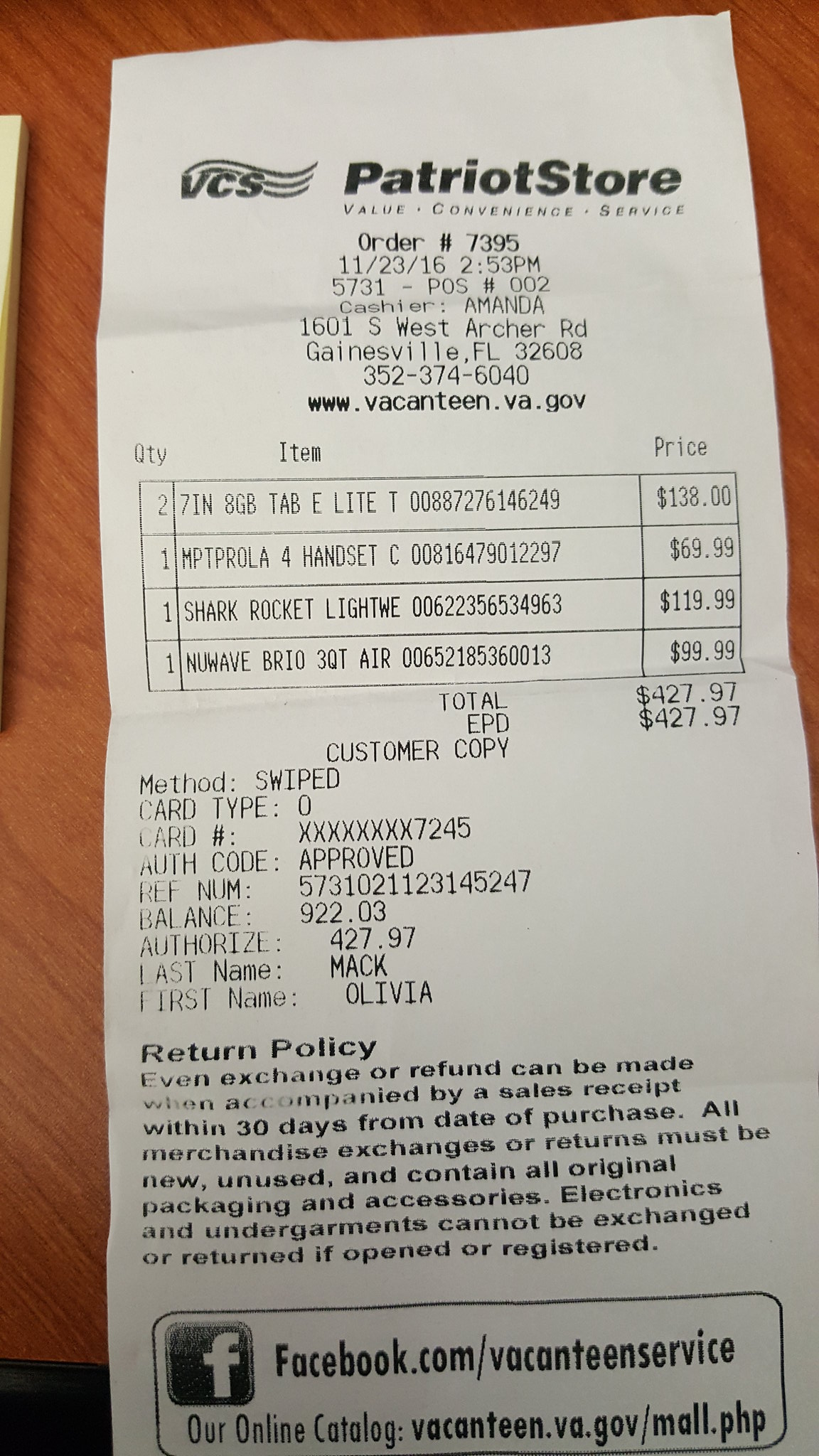The image depicts a black-and-white receipt printed on heat-sensitive paper from the UCS Patriot Store, located at 1601 SW Archer Road, Gainesville, FL 32608. The store's contact details include the phone number 352-374-6040 and the website www.vacantine.va.gov. The top section of the receipt features a logo with curved stripes beside the text "VCS Patriot Store: Value, Convenience, Service," and below that, an order number 7395-1123-16-253PM. The transaction was processed at POS number 5731-POS002 by cashier Amanda. The receipt lists four items purchased: an 8GB Tab Elite, a handset, a Shark Rocket Lightweight, and a New Wave Brio 3-quart air, amounting to a total of $427.97. The bottom of the receipt includes the last four digits of the credit card and the return policy. Additionally, there are references to a Facebook profile and several detailed line items on the purchase, such as prices $138.00, $169.99, $119.99, and $99.99.